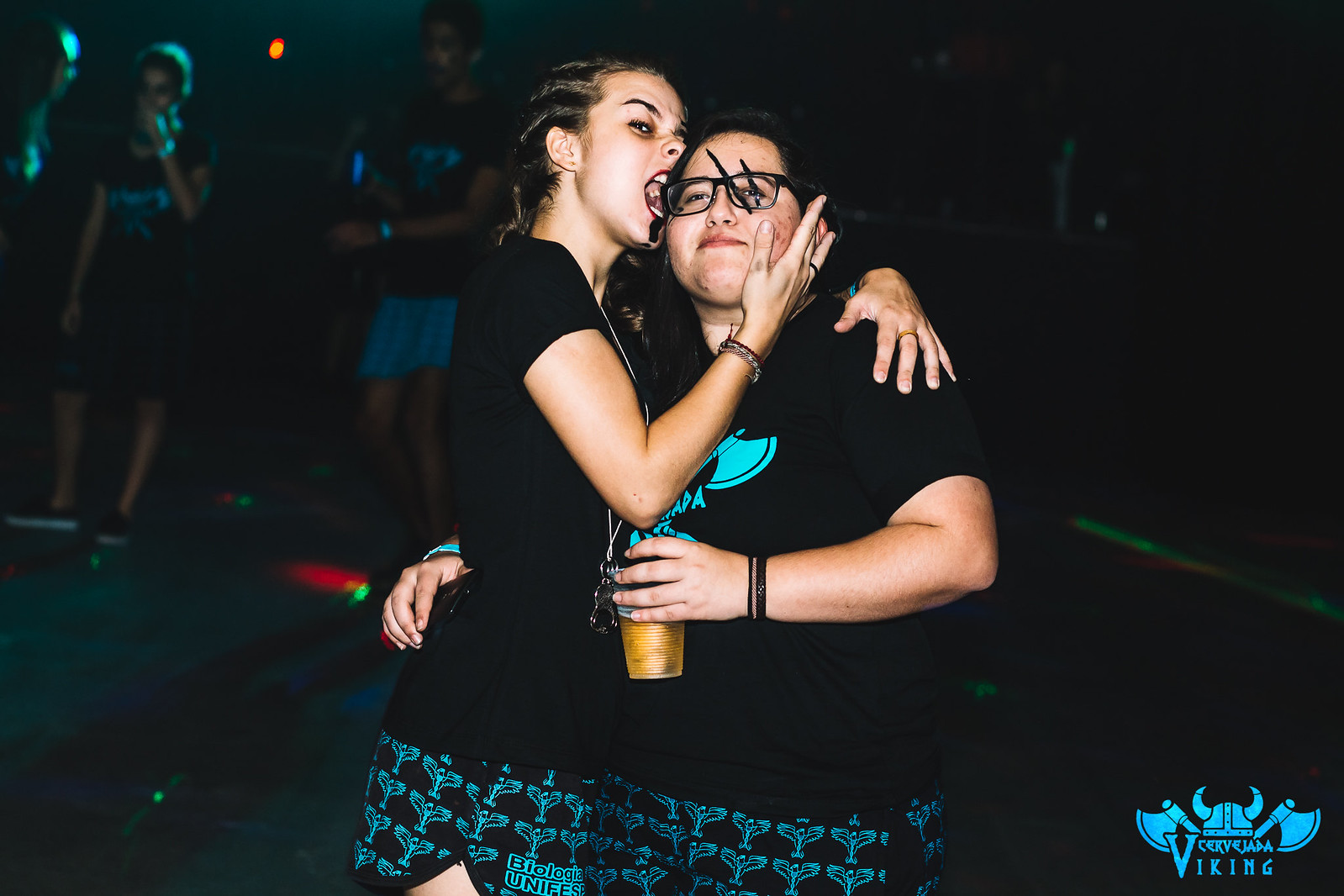In a lively and playful photograph set in a dimly lit, indoor environment reminiscent of a bar, two young women in their early twenties are captured sharing a goofy moment together. Both are attired in matching turquoise and black outfits, complete with black t-shirts featuring a distinctive Viking logo in turquoise, which is repeated on their shorts. The woman on the left, sporting glasses and face makeup mimicking a claw mark across her eye, holds a plastic cup of beer in one hand while embracing her friend with the other. Her friend, dressed identically, has her mouth open in a humorous gesture as if she is biting the other’s face. The blurred background suggests a bustling atmosphere with other people present. In the bottom right corner of the image, a logo comprising a Viking helmet flanked by crossed axes can be seen, along with the text "Cervejada Viking," hinting at an event or venue possibly themed around Viking traditions or perhaps even an axe-throwing competition. The convivial and light-hearted energy of the scene is palpable, highlighting the camaraderie and enjoyment of the participants.